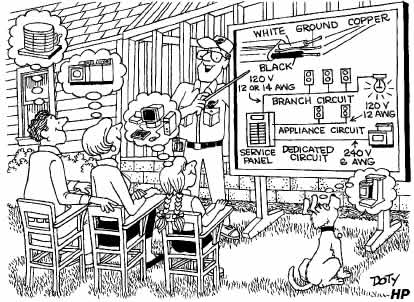In this detailed black and white single-panel cartoon strip, an enthusiastic electrician stands in front of a quaint wooden house, educating a family about electrical circuits. He is donned in an electrician's uniform, complete with a jumpsuit, hat, and glasses. The well-organized scene features the family seated attentively at desks outdoors, facing a chalkboard on legs with a drawn flowchart showcasing terms like "white ground," "copper," "120 volts," "branch circuits," "appliance circuits," "dedicated circuits," and "service panel."

Above their heads, thought bubbles reveal their daydreams about how they might use the circuits being discussed. The father envisions a central air unit, the mother imagines a washer and dryer, and the child dreams of an elaborate computer system for gaming. Even the family dog participates, fantasizing about an electric can opener for his meals. The scene humorously captures the family’s varied priorities while the diligent electrician imparts practical knowledge on home electricity.